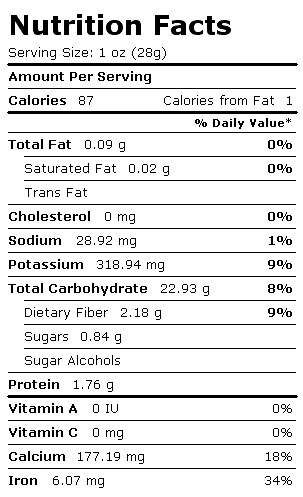The image features a standard nutrition facts label that complies with FDA regulations. The serving size is listed as one ounce, with each serving containing 87 calories, of which only 1 calorie is derived from fat. The total fat content is minimal at 0.09 grams, including 0.02 grams of saturated fat. The product contains no cholesterol and has 28.92 milligrams of sodium. Potassium content is relatively high at 318.94 milligrams. The total carbohydrate content is 22.93 grams, which includes 2.18 grams of dietary fiber and 0.84 grams of sugars. There are 1.76 grams of protein per serving. The label indicates the product does not provide any Vitamin A or Vitamin C, but it does contain 177.19 milligrams of calcium and 6.07 milligrams of iron. Given the nutritional profile, particularly the carbohydrate content, the product appears similar to chips or a similar snack food.